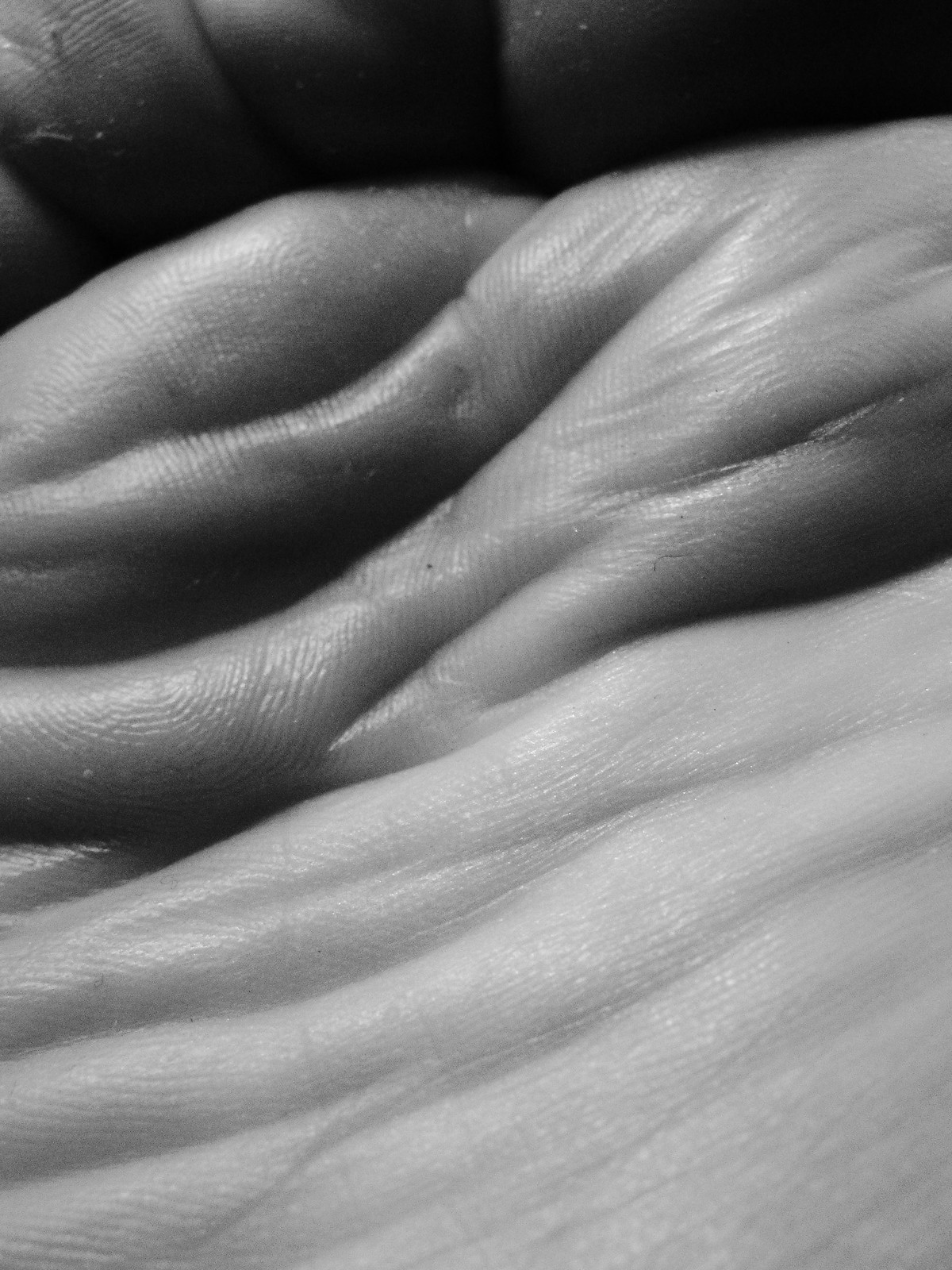The image features an extreme close-up of human skin, captured in a black-and-white photograph. The texture and lines are prominently visible, highlighting the wrinkles and slight folds in the skin. The photo's high contrast, especially with a dark-shaded area at the top, makes it hard to pinpoint the exact body part, though it most likely depicts the bottom of a foot due to the texture and prints that suggest gripping capability. A few specks of dirt are visible, hinting that the subject might be a foot. The skin appears to be smooth and healthy, belonging to a light-skinned individual. The absence of scale adds to the ambiguity, making the surface look like a complex, wrinkly landscape. The black background further isolates the skin, making its lines and textures even more stark.